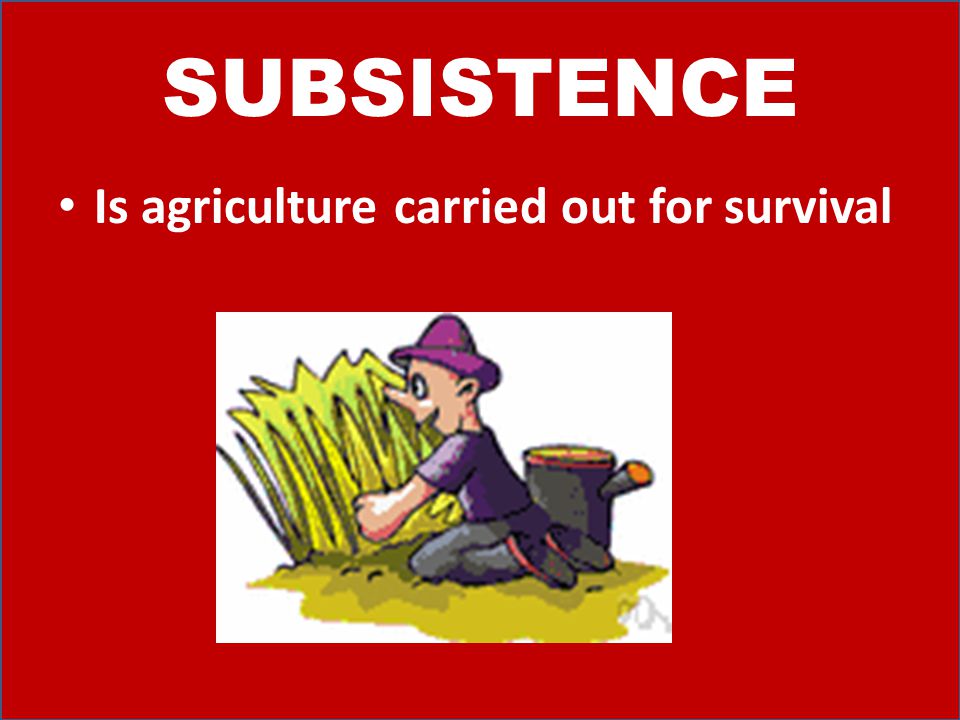The image is a horizontally oriented rectangular poster with a bright red background and white text. At the top, in very large, bold letters, it says "Subsistence." Below this, in smaller text and preceded by a bullet point, is the definition: "Agriculture carried out for survival." The bottom portion of the poster features a white rectangular box containing a low-quality, digitally created cartoon of a man kneeling on the ground, which appears to be dirt or a green surface. The man is interacting with a plant—possibly grass—while beside him sits a sizable watering can. He is dressed in gray (or black) pants, a darker purple shirt, and a purple hat. The overall layout and style suggest it could be part of a presentation slide, possibly created in PowerPoint, using a palette of colors including red, white, purple, gray, green, tan, yellow, and black.